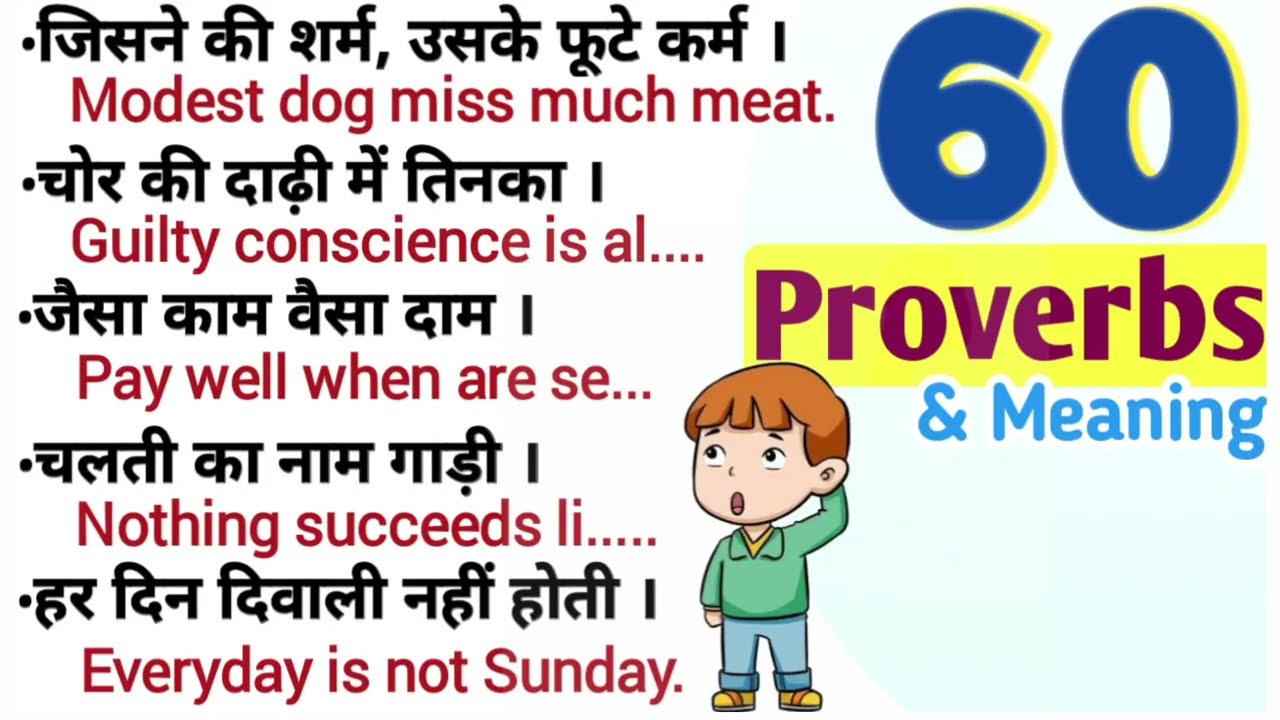This image, likely a screenshot from an app or a page from a cartoon or book, prominently features the title "60 Proverbs and Meaning." At the top right corner, the number "60" is displayed in large blue text with a yellow border. Below this, a yellow rectangle contains the word "Proverbs" in dark reddish-purple, and beneath it, "And Meaning" is written in blue.

The background of the image is white, and the main section on the left side is occupied by vertical rows of black text in an Arabic script. Directly beneath each Arabic proverb, translations in red English text read: "Modest Dog Missed Much Meat," "Guilty Conscience Is, A-L," "Pay Well When R-S-E," "Nothing Succeeds, L-I," and "Every Day Is Not Sunday."

In the bottom center, there's a cartoon character of a small boy with short brown hair and pale skin, wearing a long-sleeved collared green shirt, blue jeans, and brown shoes. The boy stands with one arm behind his back and the other hand behind his head, appearing surprised. This childlike figure adds a playful touch to the educational nature of the image.